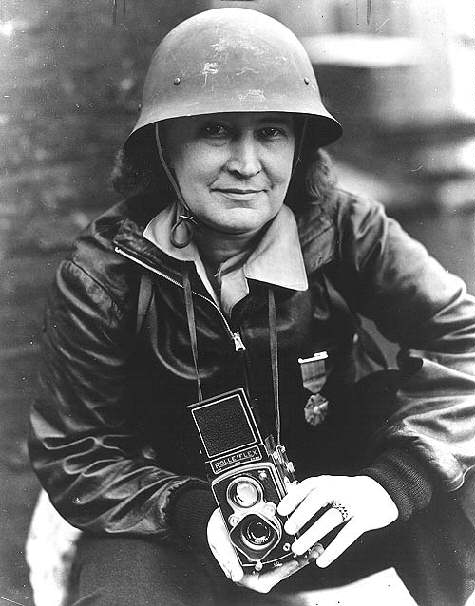This black-and-white portrait captures an older Caucasian woman, likely in her 40s or early 50s, seated on a white chair with a blurred background. She appears to be a wartime reporter, given her attire – a military hard hat with a chin strap and a black leather bomber jacket zipped up to her chest, under which she wears a collared shirt. Her dark hair falls just above her shoulders. 

The woman wears a notable patch on her jacket along with a metal pinned on her left side. She is holding an old-fashioned box camera – possibly a Roloflex or Holoflex – with a strap around her neck. Both of her hands grasp the camera, and on the ring finger of her left hand, she wears a band. Her posture is slightly relaxed, sitting with her left knee more bent than her right, her forearms resting on her thighs. The image suggests a sense of historical significance, capturing a moment that blends the military and journalistic essence vividly.